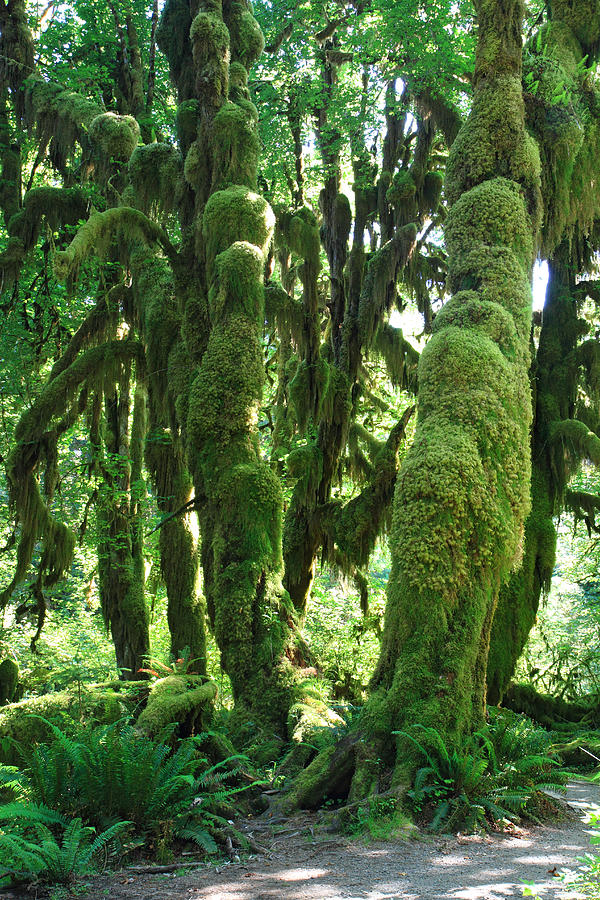In this vibrant daytime photograph of a unique forest setting, lush green moss blankets nearly every visible surface of the tree trunks and branches, effectively obscuring most of the bark and creating an almost otherworldly atmosphere. Sunlight filters through the dense canopy, casting radiant reflections upon the verdant grass and bushes below. Fleeting glimpses of a clear blue sky appear through separations in the tree branches above, enhancing the scene's ethereal beauty. In the bottom left corner, a bush stands amidst a scatter of gravel and rocks, indicating a worn path or trail. This pathway, strewn with small pebbles and natural debris, meanders to the right, inviting deeper exploration into the moss-clad, fern-draped landscape. The forest floor is a lush carpet of green plants, and the tendrils of moss, hanging from the branches and climbing the tree trunks, lend a mysterious, almost creepy aura to the scene. The overall impression is one of dense, thriving greenery in a setting reminiscent of a tropical or subtropical environment.